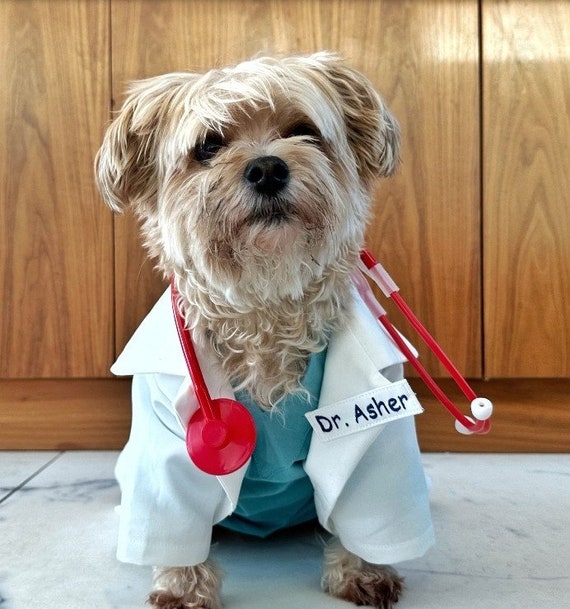This adorable photograph captures a small, light tan dog dressed as a doctor. The dog, resembling a breed similar to a Toto-like canine but lighter in color, sits alert on a marble-tiled floor against medium brown, grainy wood paneling. He's dressed in a white doctor's coat with a green V-neck scrub top underneath. A bright red plastic stethoscope with white ear tips hangs around his neck, and a name tag reads "Dr. Asher." His fluffy ears hang down, and some of his fur falls over his dark eyes, adding to his cute, attentive expression as he looks slightly upwards, possibly waiting for a treat.